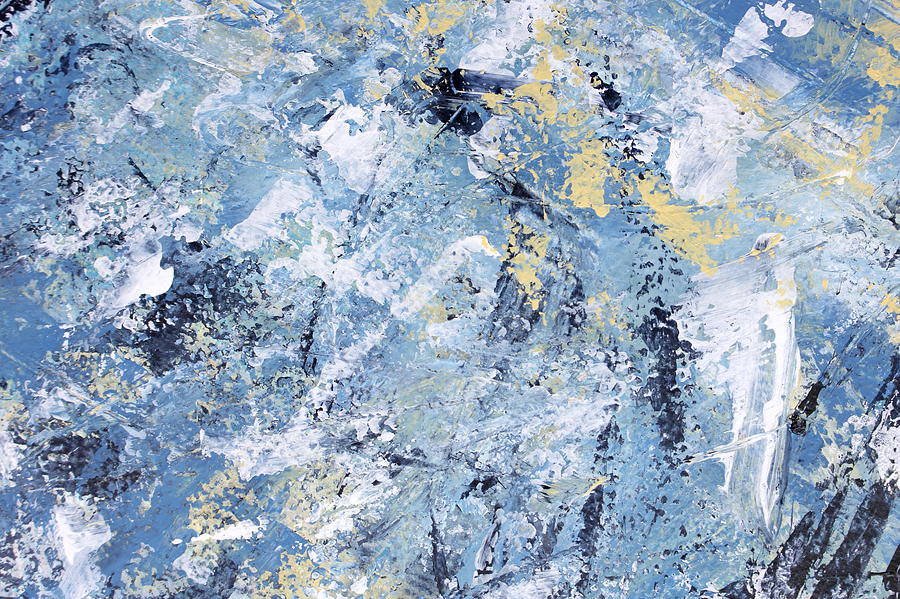The image depicts an abstract painting that appears to be created with acrylic or oil on canvas. The artwork features a primary color palette of various shades of blue, ranging from light to dark, and is complemented by white, black, light brown, and pale butter yellow splotches. The composition is haphazard, with colors seemingly thrown at the canvas or smeared across it in a disorganized fashion, creating random patches, splatters, and jagged areas. The blue tones dominate the background, giving the impression of an ocean from a distance, while the lighter and darker shades, along with other colors, add depth and texture. The thick application of paint in certain areas suggests the use of a trowel or scraper to create the textured effect, resulting in an overall visually striking and chaotic blend of colors that forms an intriguing abstract piece.